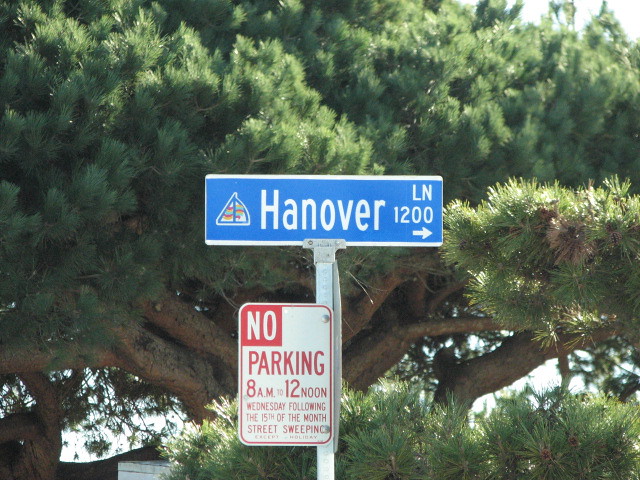This horizontal, rectangular photograph features a blue street sign with white borders situated against a lush backdrop of green trees. The sign prominently displays the place name "Hanover" in bold white letters, with a stylized, cartoony sailboat logo depicted in white to the left of the text, hinting at a coastal or beachside location. To the right, it indicates "LN 1200" with a white arrow pointing right, possibly signifying a direction or distance. Below the Hanover sign, a white and red bordered no parking sign details regulations: "No Parking 8 AM to 12 Noon, Wednesday following the 15th of the month, Street Sweeping." The background is filled with thick-branched trees with abundant green leaves, and glimpses of blue sky peek through the foliage, adding a touch of serenity to the setting.